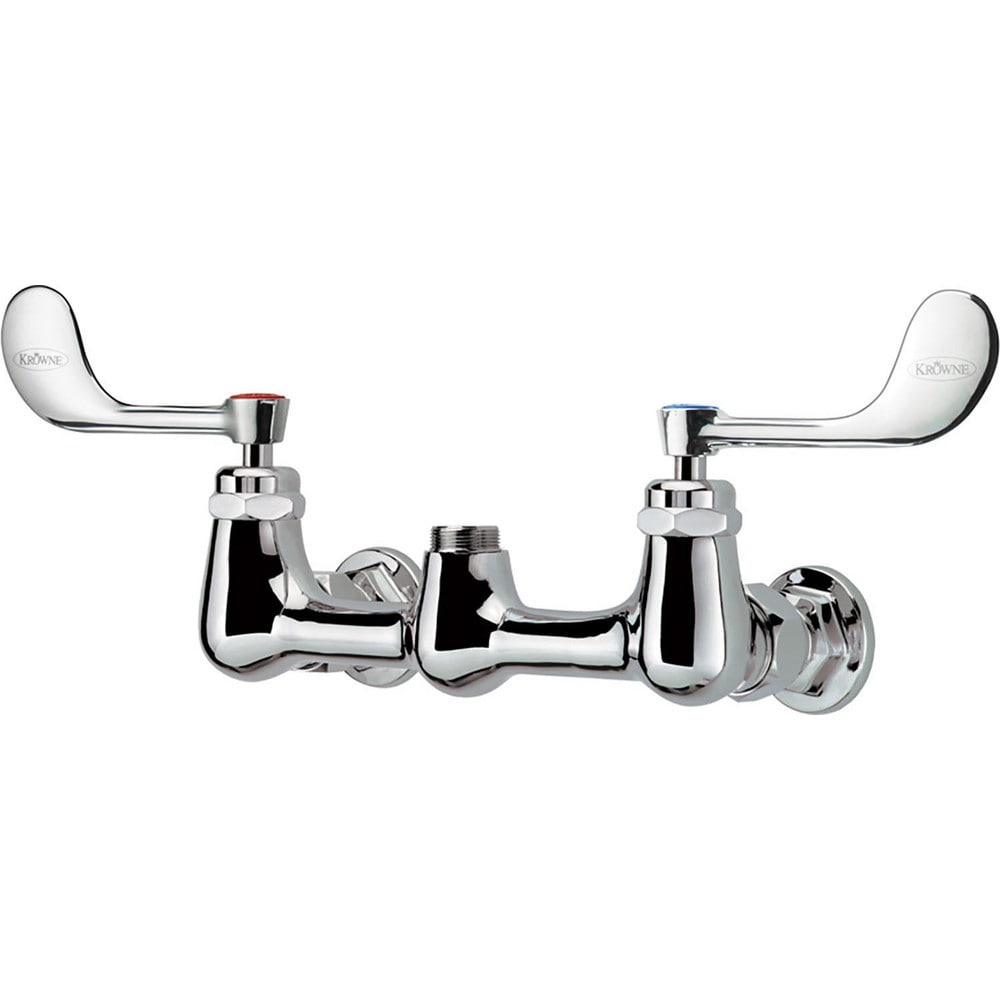This photograph features a close-up view of a faucet assembly set against a pure white background. Central to the image are two shiny, brand-new handles made of what appears to be stainless steel. The handles, positioned on the left and right, are designed to turn inward—left handle towards the right and right handle towards the left. In the center, where these handles connect, there is a fitting for a water spout, though the spout itself is not attached and would need to be screwed in manually. 

The left handle is distinguished by a red tab indicating hot water, and the right handle by a blue tab indicating cold water. Each handle bears a logo with the brand name "Krowne" (spelled K-R-O-W-N-E), featuring a notable crown above the letter "O" set within an oval sketch. This logo is printed in small text and appears on the end of both handles. The faucet handles, overall, give off a sleek and modern look with additional black trim elements. 

This detailed representation highlights both the functional and aesthetic aspects of the faucet set, emphasizing its fresh, polished appearance and clear distinction between hot and cold water controls.